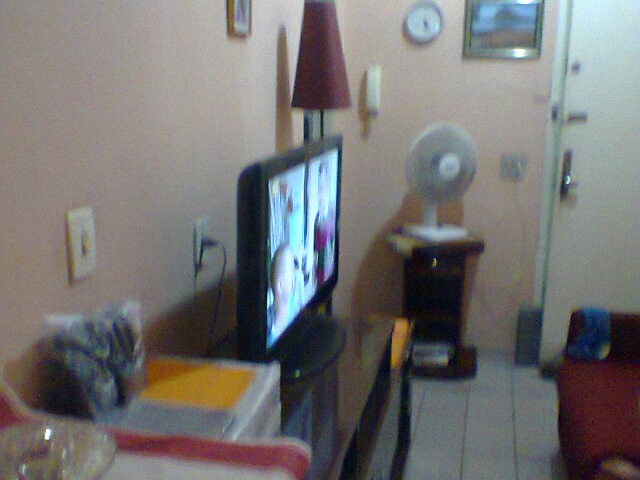The image depicts a small, somewhat cluttered room that resembles an apartment or possibly a hotel room. The focal point is a television with a black border that is turned on, displaying a program with predominantly blue and purple hues. The television sits on a wooden stand, which also holds additional items. A white tile floor with grey molding is visible, adding to the room’s clean, albeit compact appearance.

To the left of the television, there is a small white fan on a stand, situated under a picture and a round clock displaying the time around 6:25. A lamp with a red shade stands in the corner, parallel to a tan-colored door that has a chain lock and a metal handle. This door contrasts with the walls, which are of a white-pinkish hue, lending a soft pastel tone to the room.

A red chair, upholstered and partially obstructed from view, has something blue draped over its right arm and faces the television. A cellophane package with a dark object inside sits on a counter in the foreground, near a light switch. The image, slightly blurry, reinforces the cozy yet utilitarian feel of the space, with no people present in the scene.